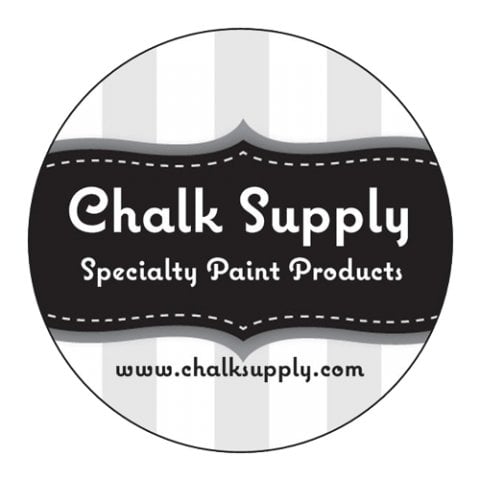The image is a black and white advertisement featuring a large circular design with light gray and white vertical stripes. The circle is bordered at the top and bottom by wavy gray lines, which add to the decorative element. Across the center of the circle is a horizontal black banner with white text that reads "Chalk Supply," with "Chalk" in a cursive-like font and "Supply" in a slightly curvy print. Just below this, also in white text but in a smaller, clear font, it states "Specialty Paint Products." Further down, in even smaller text, the website "www.chalksupply.com" is displayed. The overall layout is clean and legible, emphasizing the brand name and product line against the contrasting black background.